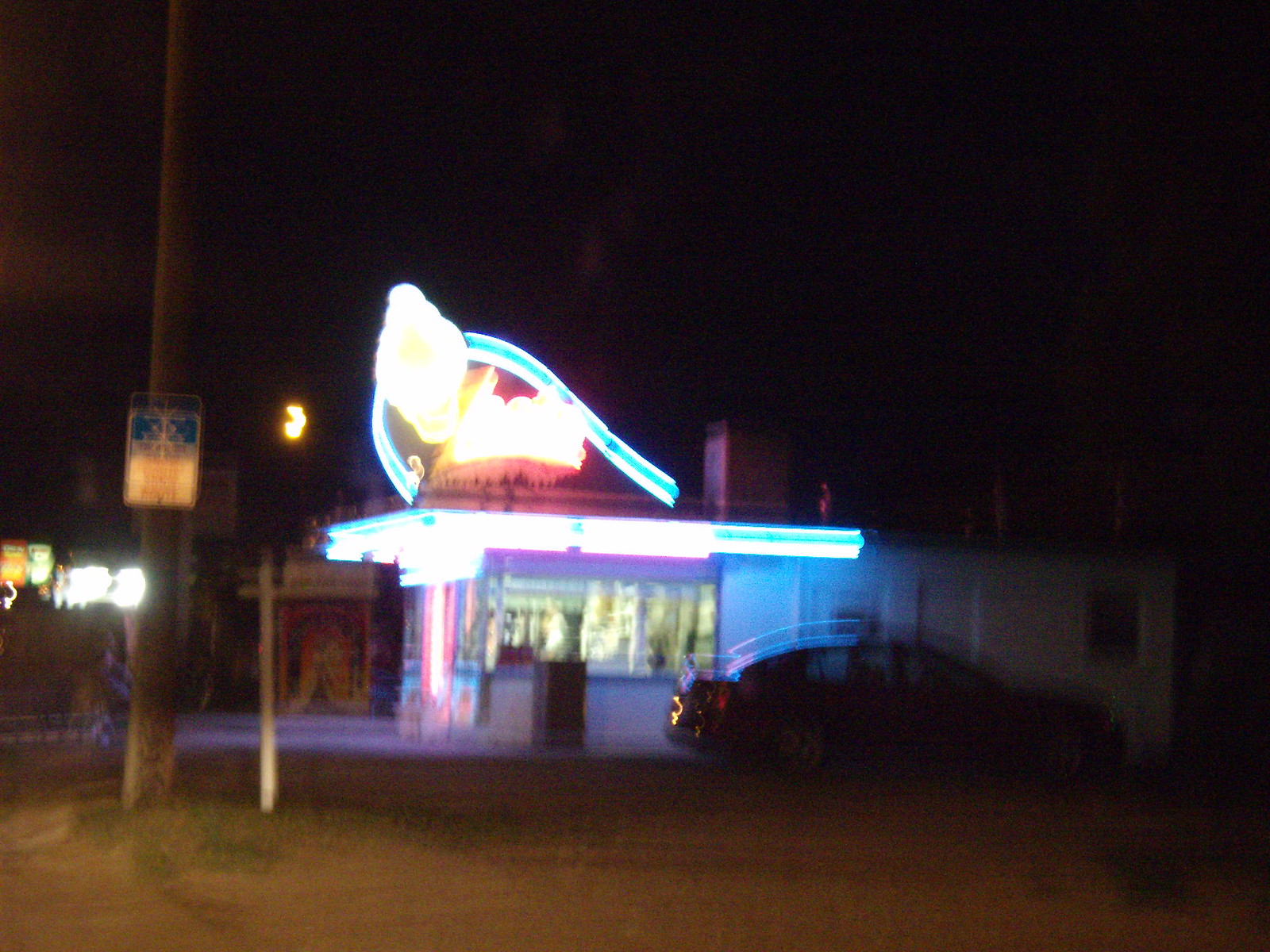A blurry, color photograph taken at night captures the vague outline of a car parked in a shadowy area. The car is situated in a dimly lit lot, presumably in front of a building that seems to be a restaurant. The building is adorned with a bright, round fluorescent sign, which is overexposed and has a blue edge with an indistinct round object in the center. Below the sign, the roof glows with fluorescent light, spilling pink and blue hues around the windows beneath it. To the left side of the image, a tall pole holding a blue and white sign stands alongside a smaller pole. Additional street lighting illuminates the very left-hand corner of the scene. The night sky is almost pitch black, with a tiny patch of grass visible under the street signs on the ground.